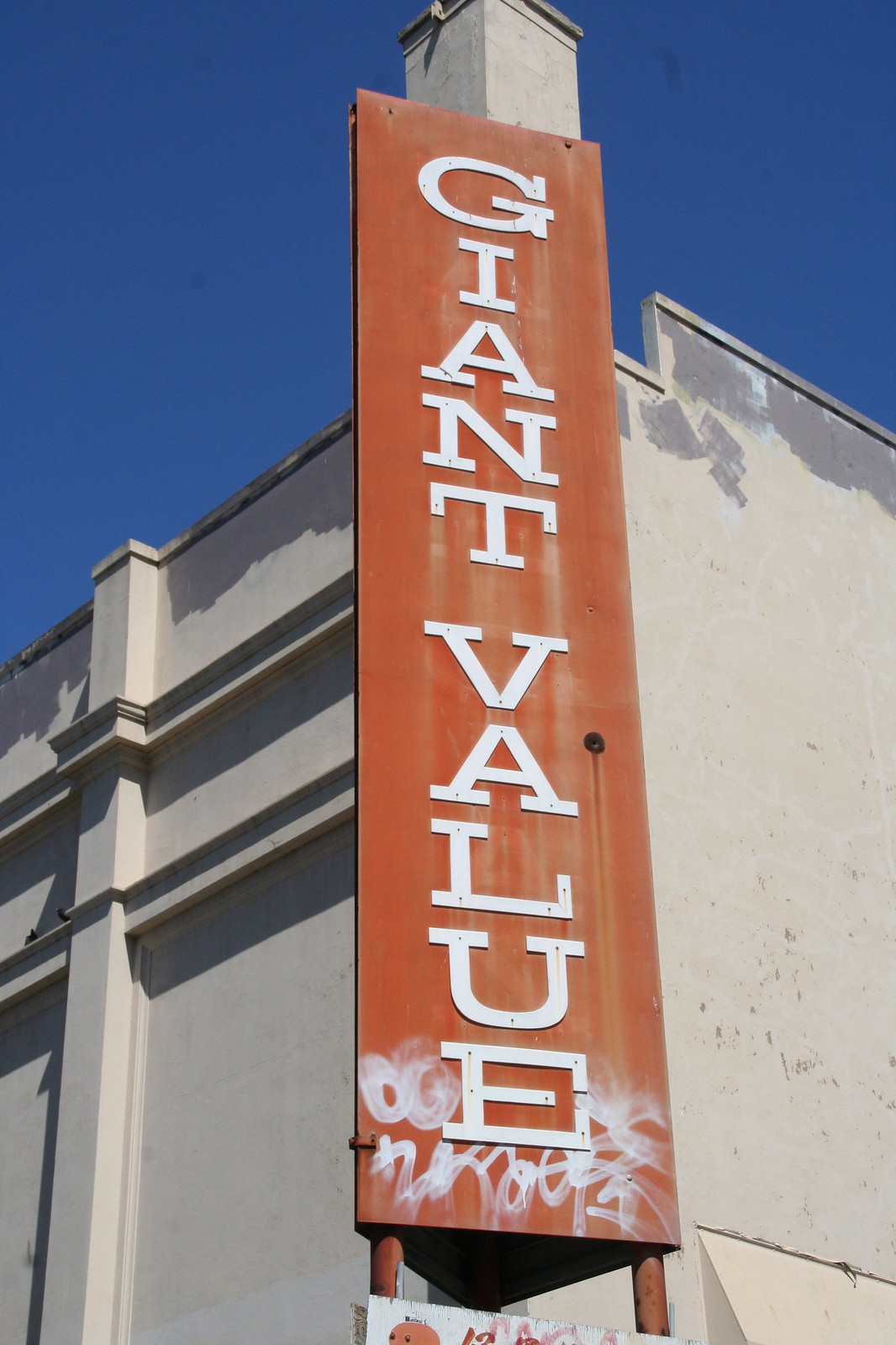This image captures the upward view of the beige corner of a building against a clear, blue sky. Dominating the scene is a vertical, red rectangular sign reading "Giant Value" in bold, white block letters. The sign shows signs of age and weathering, with faded sections and graffiti in white spray paint near its base. On either side of the building’s top corner, there are gray splotches. Additionally, just below the red sign, the upper edge of a white sign is visible, though its details are obscured.